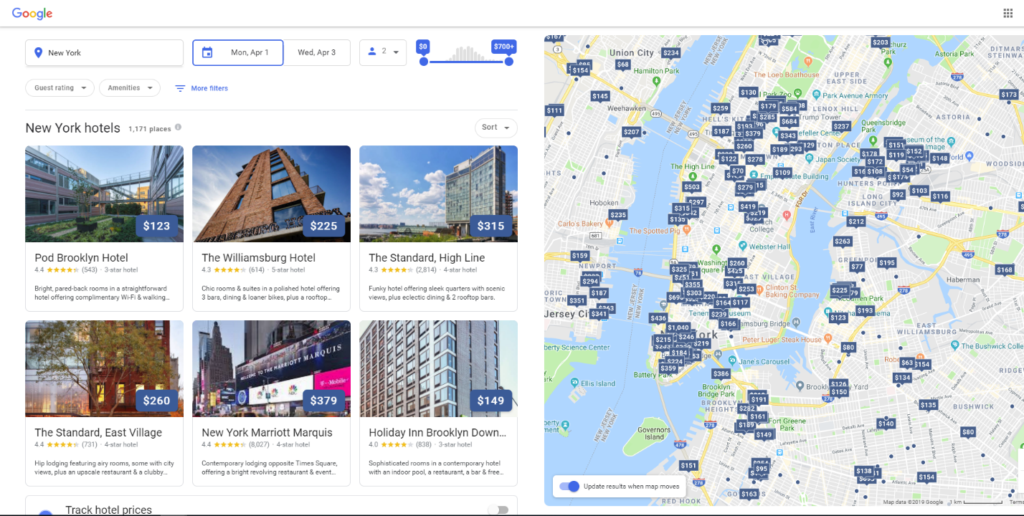The image is divided into two sections. The left side features a series of images and text, while the right side displays a detailed map. On the left, the word "Google" is presented in vibrant rainbow colors. Below it, there are six tiles showcasing various hotels, each marked with a small blue rectangle indicating prices in white text. 

One of the hotels is a tall structure, predominantly composed of windows, with a backdrop of a bright blue sky and scattered white clouds. Another hotel is characterized by its brown brick facade and yellow windows, accompanied by a tree in the foreground and labeled "The Standard East Village." Scattered across these tiles are several yellow stars, likely indicative of the hotels' ratings.

The right side of the image is occupied by a map, crisscrossed with yellow lines representing roads. Among these roads are multiple blue rectangles with prices in white text, mirroring the style on the left. The map also includes blue areas symbolizing bodies of water. In the top left corner of this section, there's a location marker with a text box containing the word "New York." Additionally, an icon of a calendar is present next to the text "MON, April 1," with the box outlined in blue, possibly indicating a specific date for bookings or events.